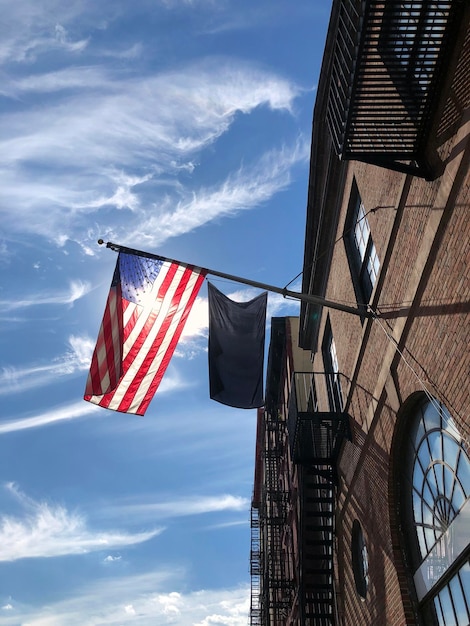The photograph captures the perspective of someone standing at the base of a tall, dark red brick building, looking upwards towards the sky. The building, which could be a bank or a stately apartment, exhibits a mix of red, tan, and black bricks, and features several architectural details including a fire escape, metal-barred balconies, and windows with decorative crossboards forming a starburst effect. The sky occupies around 60% of the image and is a clear blue with a few wispy white clouds. Prominently displayed at the top of the building is an American flag, extended to the left on a flagpole. The flag partially obscures the sun, causing its stars and stripes to be dramatically illuminated. Another, unidentified dark flag can also be seen, though it is less prominent. The overall impression is one of urban architecture accented by a patriotic symbol, with the sky and flag creating a compelling focal point against the structured backdrop of the building.